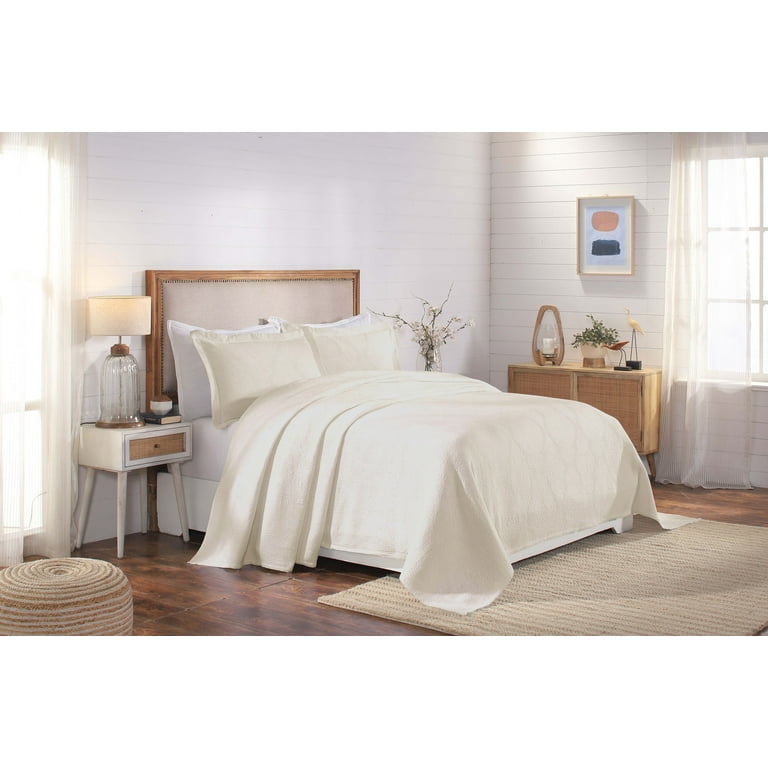This is a horizontal-rectangular photograph of a beautifully decorated bedroom, characterized by its predominantly white color scheme. The white walls are adorned with two large windows covered in sheer white drapes, one extending to the floor. Centrally positioned is a full-size bed featuring an elegant sleigh headboard with white fabric in the center and a brown wooden rim. The bed is dressed in an off-white spread with two matching pillows, two additional white pillows, and a cream-colored blanket. 

Flanking the bed are two nightstands; the one on the left holds a lamp with a white lampshade, while the right one has a vase of artificial flowers. A small brown dresser, topped with two candles, a small bucket of greenery, and another lamp, stands against the opposite wall. Above it hangs a photograph with a mixture of pink and green colors. At the foot of the bed, a beige carpet lies over a dark wood floor, partially covering an ottoman. This serene and minimalist room also features a small cabinet below the photograph and a beige footstool, completing the cozy yet elegant aesthetic.